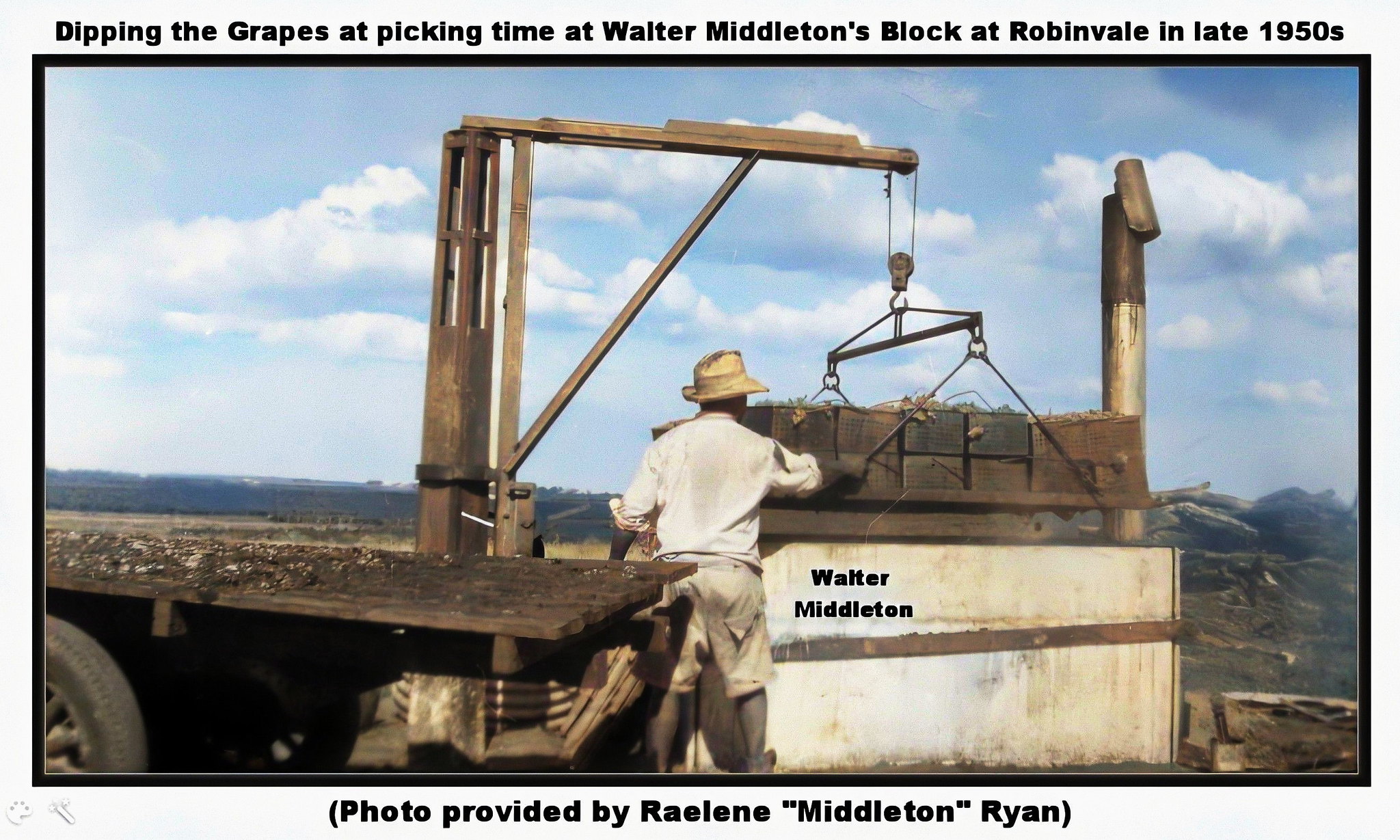The image features a historical photograph framed by a light gray border. The text on the top and bottom of the border reads, "Dipping the grapes at picking time at Walter Middleton's block at Robinvale in the late 1950s. Photo provided by Raylene Middleton Ryan." At the center of the image stands Walter Middleton, identifiable by the black text next to him. Middleton, a black male, is facing away from the camera, wearing light-colored shorts, a light long-sleeved top, and a straw hat. He is outdoors, in what appears to be a farm setting on a sunny day, possibly midday. To his left is a flatbed trailer made of wood with visible tires at the bottom left corner. Attached to or situated behind the trailer is a hoist mechanism with a pulley system lifting a pallet loaded with several dark-colored boxes. Walter Middleton is seen operating or steadying this machine. The overall color palette of the photograph includes shades of light gray, black, light blue, white, gray, and brown. The backdrop reveals an open sky, emphasizing the outdoor rural environment.